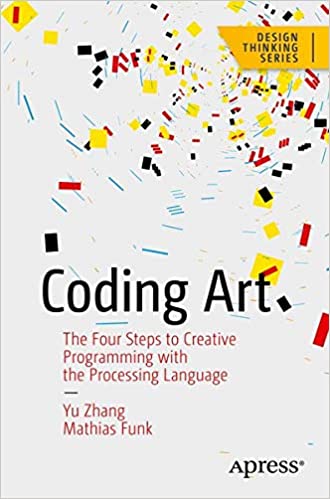The cover of the book "Coding Art: The Four Steps to Creative Programming with the Processing Language" by Yu Zhang and Matthias Funk features a dynamic and visually intricate design. Against a white background, the cover showcases a vibrant vortex of swirling shapes, including yellow squares, black and red rectangles, and thin blue rectangles, all varying slightly in size. The vortex is centered near the top right of the cover, creating a sense of movement and energy. At the top right corner, a yellow ribbon with black text reads "Design Thinking Series," accompanied by a vertical black line. In the top left corner, there's a tilted yellow square placed diagonally like a diamond. The title is prominently displayed in large black letters near the center, with the subtitle in smaller red font beneath it. The authors' names are also featured beneath the subtitle. At the bottom right corner, the publisher's name, A Press, is printed in black. The overall design is enhanced by confetti-like pieces swirling around, adding to the cover's lively and creative aesthetic.